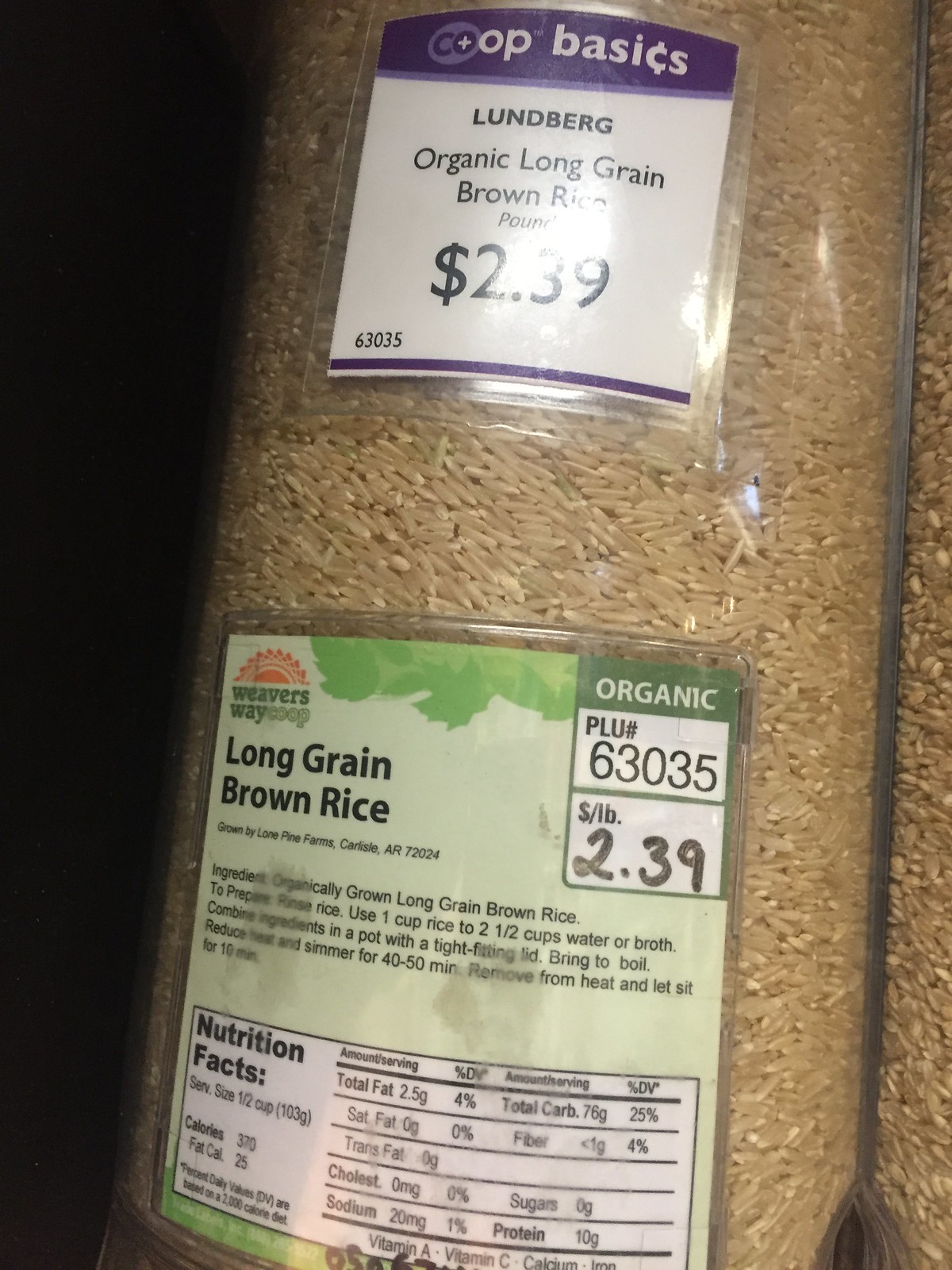This image is a portrait-format, color photograph of a bulk bin containing organic long grain brown rice. The bulk bin appears to be made of plastic, featuring a horizontal silver rod, and it has two labels displayed on it. The top label is white with a purple top and bottom border, labeled "Co-op Basics Lundberg Organic Long Grain Brown Rice, $2.39 per pound, PLU 63035." The bottom label is light green with green borders, containing a logo of an orange sun and labeled "Weaver's Way Co-op Long Grain Brown Rice, Organic, $2.39 per pound, PLU 63035, ingredients: organically grown long grain brown rice, grown by Lone Pine Farms, Curly Seed R72024." Additionally, the label provides cooking instructions stating to rinse the rice and use one cup of rice with two and a half cups of water or broth, combining in a pot with a tight-fitting lid. Furthermore, the label includes Nutrition Facts, highlighting a serving size of half a cup. The rice itself is visibly brown, distinct from white rice.